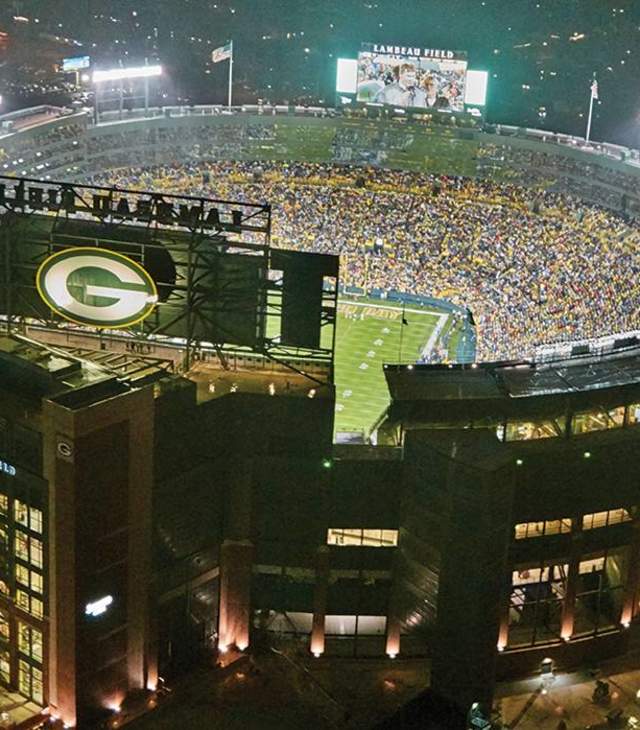This aerial view captures the bustling, electrifying atmosphere of the Green Bay Packers' Lambeau Field. Dominating the scene is a large, distinctive white "G" logo set against a green circle and encircled by a yellow border, prominently displayed on the back of a dark billboard. The open-air stadium is brimming with fervent fans, nearly every seat filled, all soaked in team colors of green and yellow. 

At the heart of the stadium, the green football field, marked with faintly visible field markers, hosts groups of players. Above the crowd, two American flags flutter proudly on tall posts flanking a massive screen, which currently features the Packers' president addressing the crowd. The illuminated Lambeau Field sign crowns the screen, which is bordered on both sides by glowing neon signs, adding to the vibrancy of the scene. Stadium lights shine brightly, piercing the night, as the spectacle unfolds within this iconic arena.